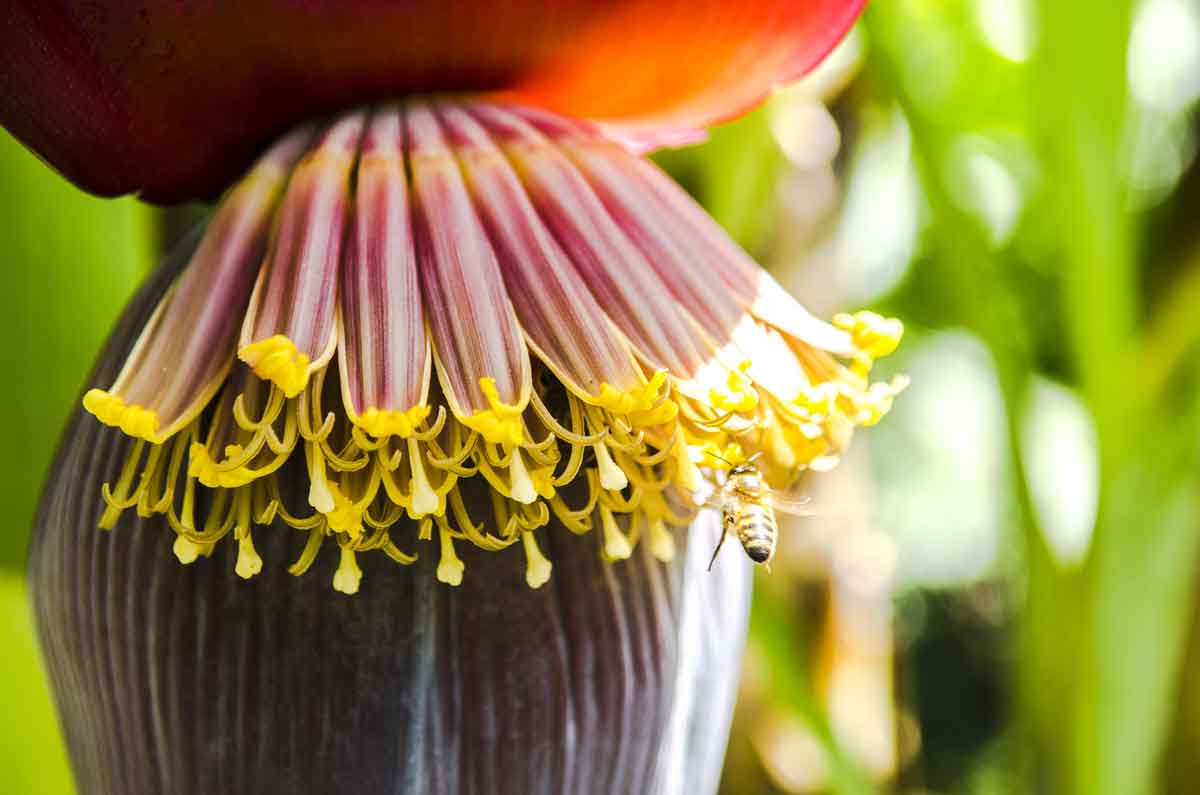The photograph is a detailed and captivating close-up shot of a large, vibrant flower with intricate features and a bee approaching it mid-flight. The image is rectangular, with the top and bottom sides twice the length of the left and right sides. In the background, mostly on the right and far left, there are multiple green plants that are out of focus, showing only their long green stems and grasses. The main flower prominently displays a bulbous, purple base leading up to a large singular petal in shades of pink and purple, pointing upwards. This petal is adorned with multiple thin, oblong purple and white petals, each tipped with a delicate white filament. There is also a honeybee with black and yellow stripes, clearly visible with its wings, two legs, antennae, and eyes, flying towards the flower, likely aimed at collecting pollen from the intricate inner parts of the bloom.